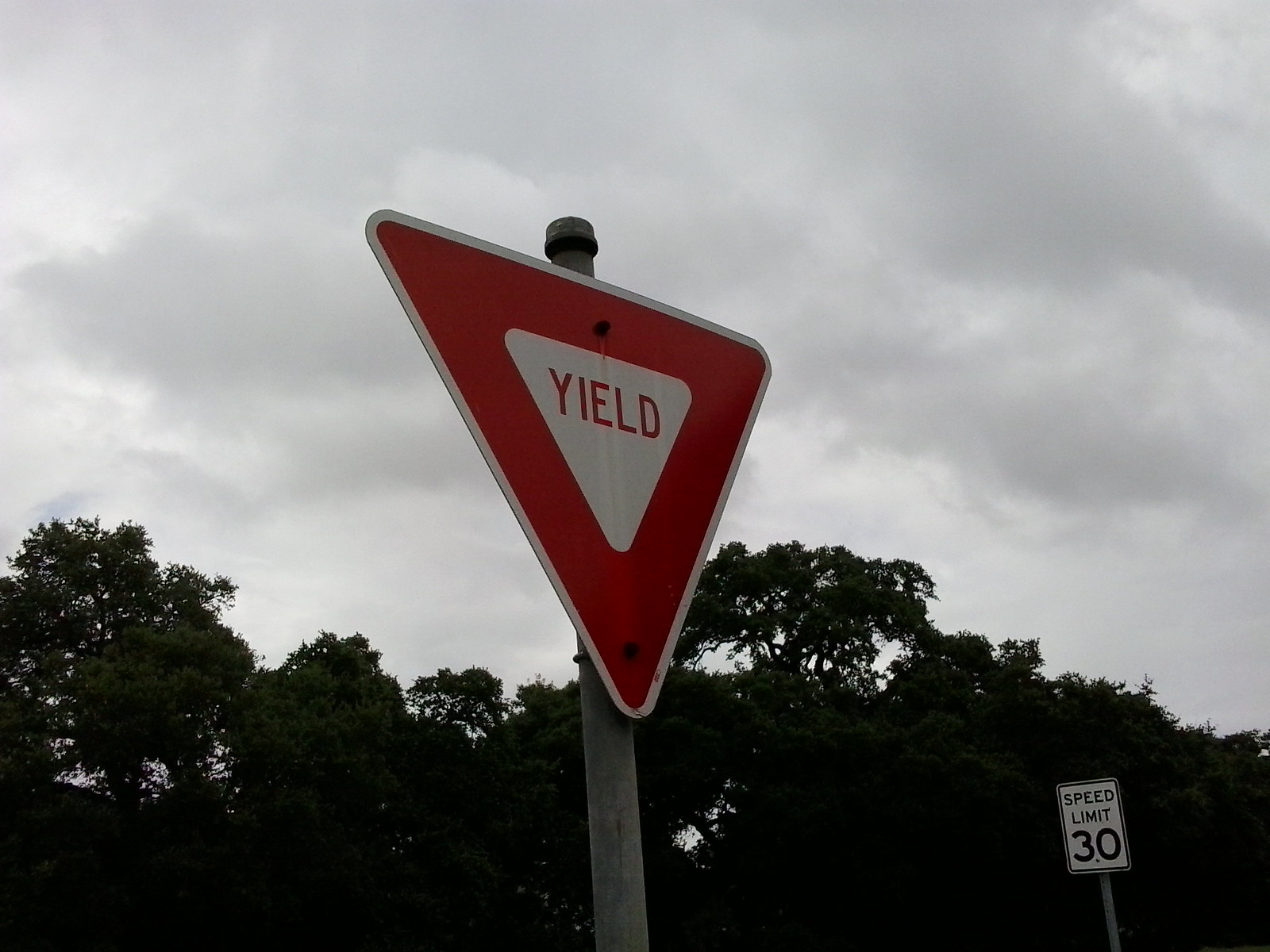This outdoor photograph, taken on a cloudy day, features a close-up of a prominently centered yield sign affixed to a silver metal pole. The sky takes up the top two-thirds of the image and is filled with gray, whitish clouds, with a possible hint of blue. The bottom third reveals dark, indistinct trees adding depth to the scene. The yield sign itself is an upside-down triangle with a bold red border, a thinner white outline encasing it, and a white inner triangle that bears the word "YIELD" in all caps written in red. To the right in the photograph, though further back due to perspective, stands a speed limit sign on another silver pole. This sign is a white rectangle outlined in black, displaying the text "SPEED LIMIT" and the number "30" below it in black lettering.